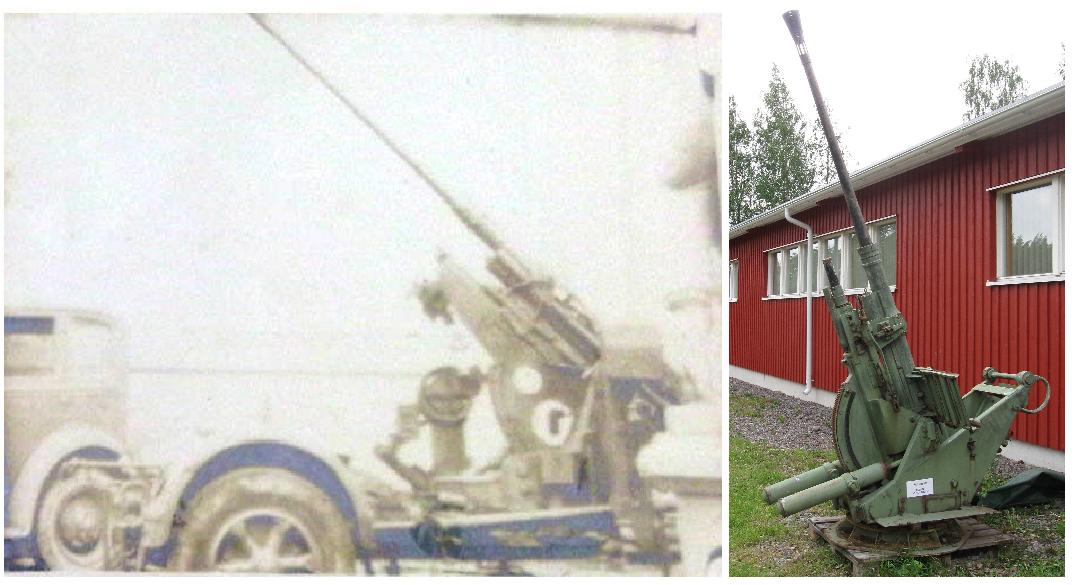The image is a composite of two photographs placed side-by-side, illustrating a stark contrast between past and present. On the left, a faded, washed-out photo or scan showcases an old World War II era anti-aircraft gun mounted on the bed of a large-wheeled truck. This historical image is in grayscale, adding to its antiquated appearance. To the right, a vibrant, modern-day color photograph captures a similar anti-aircraft gun, painted in military green, positioned outside. This cannon, with its long barrel pointed towards the sky, is set against a vivid backdrop of a single-story red house with white roofing. The scene features details like a grassy and gravel-strewn ground, overcast skies with visible clouds, and surrounding trees, firmly grounding it in a contemporary context while echoing the past.